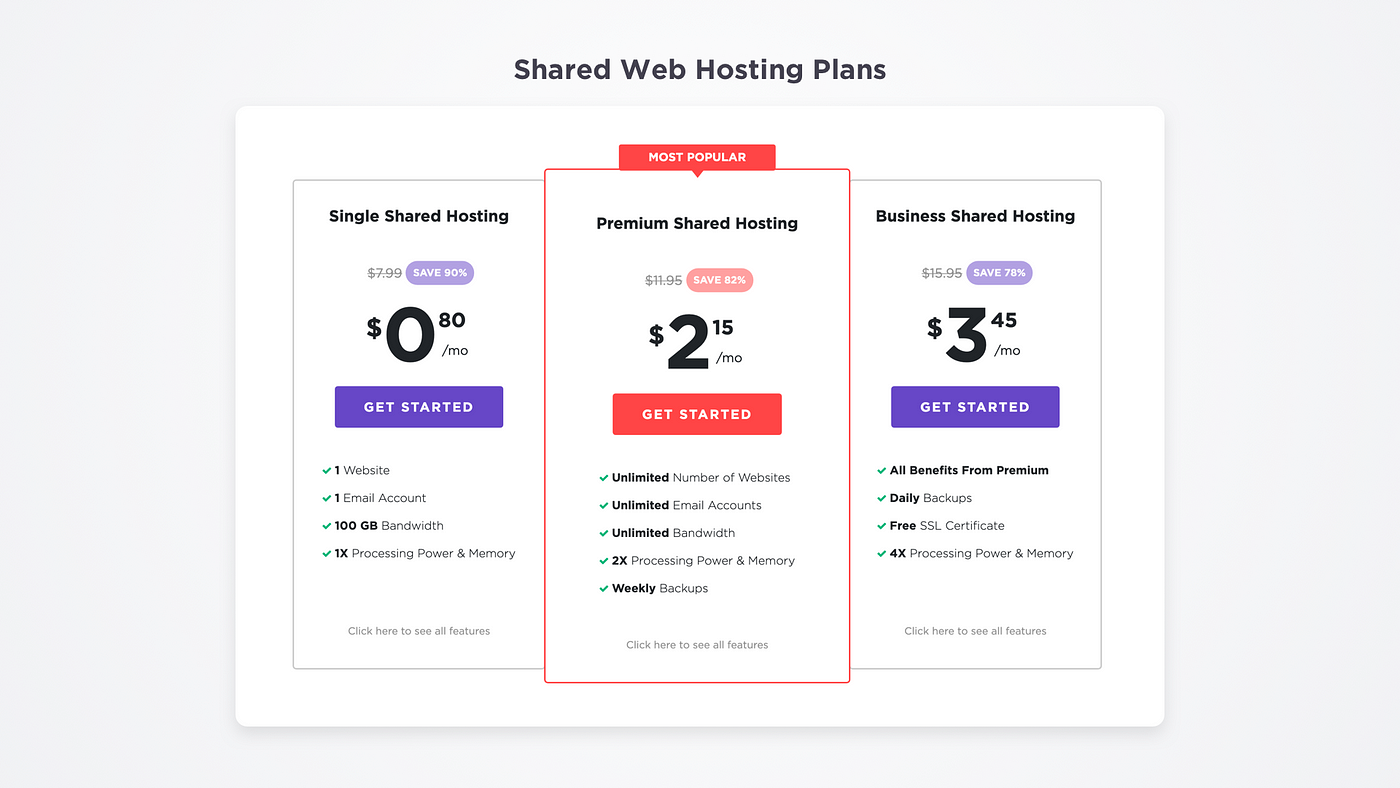The image showcases three web hosting plans against a light whitish-gray background. These plans are presented within a white box, set side by side for easy comparison. At the top of the white box, the title "Shared Web Hosting Plans" is prominently displayed in black font. 

The first plan on the left is labeled "Single Shared Hosting." It features a promotional offer to "Save 90%," with the original price of $7.99 shown in gray and crossed out. The discounted rate of $0.80 per month is displayed in a larger, bold black font.

The middle plan is named "Premium Shared Hosting" and includes an offer to "Save 82%." This option is priced at $2.15 per month.

The third and final plan on the right is called "Business Shared Hosting," offered with a "Save 70%" discount. The monthly cost for this plan is $3.45.

Overall, the image provides a clear, visually appealing presentation of different web hosting plans, detailing the savings and monthly costs for each option.